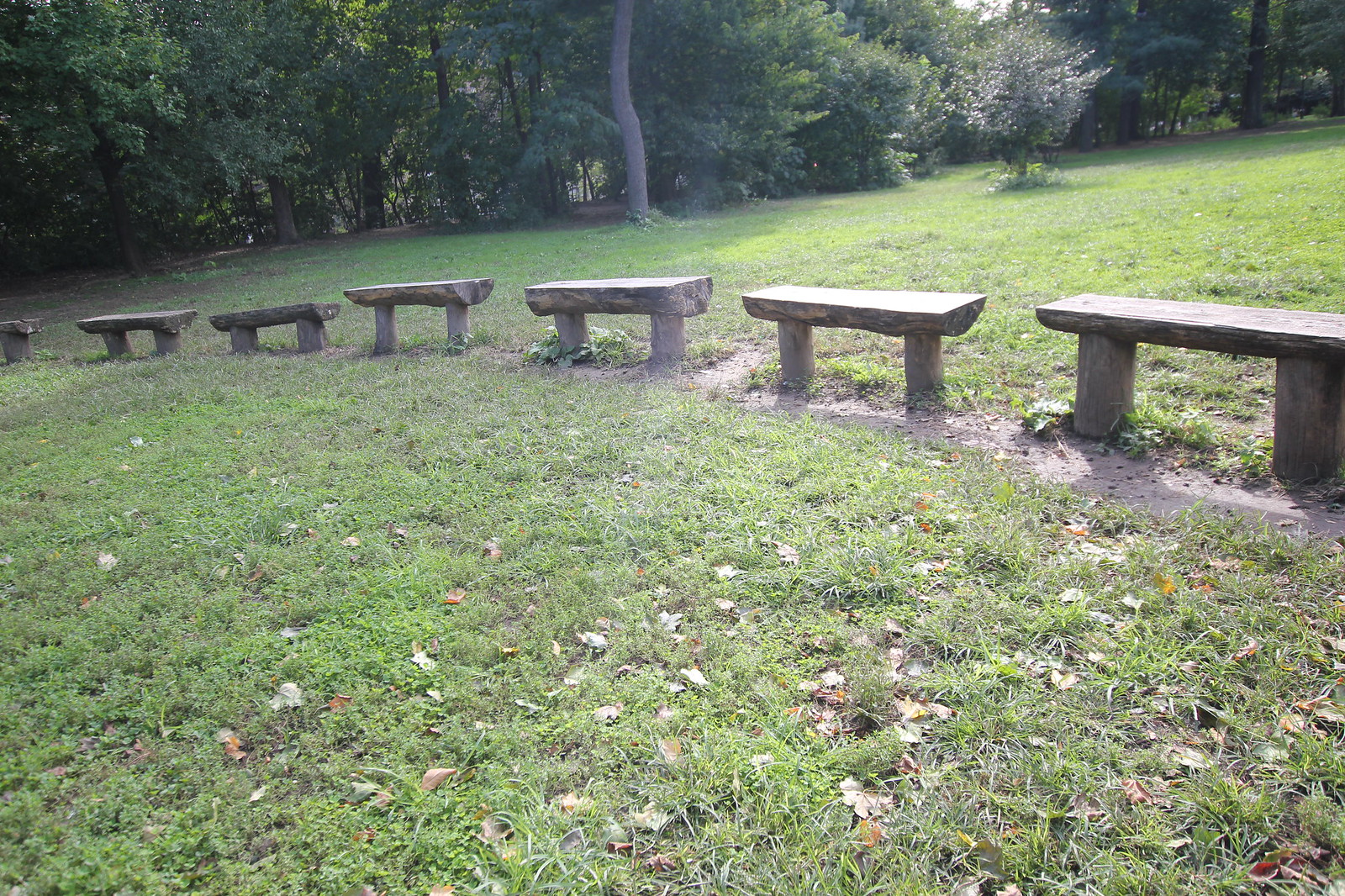The photograph captures a tranquil outdoor setting in what appears to be a secluded park or nature reserve area. The central focus is on a series of seven rustic, solid stone benches arranged in a row, each supported by two sturdy columns. They are situated on a grassy expanse speckled with scattered, dead leaves, suggesting an early autumn season. The benches' placement on the grass and dirt, devoid of any occupants, enhances the scene's sense of quietness and serenity. In the background, the gently rising landscape transitions into a small hill adorned with a variety of lush, dense trees. Sunlight filters through the trees from the upper right corner, casting portions of the scene in dappled light and shadow, further contributing to the serene and secluded atmosphere.